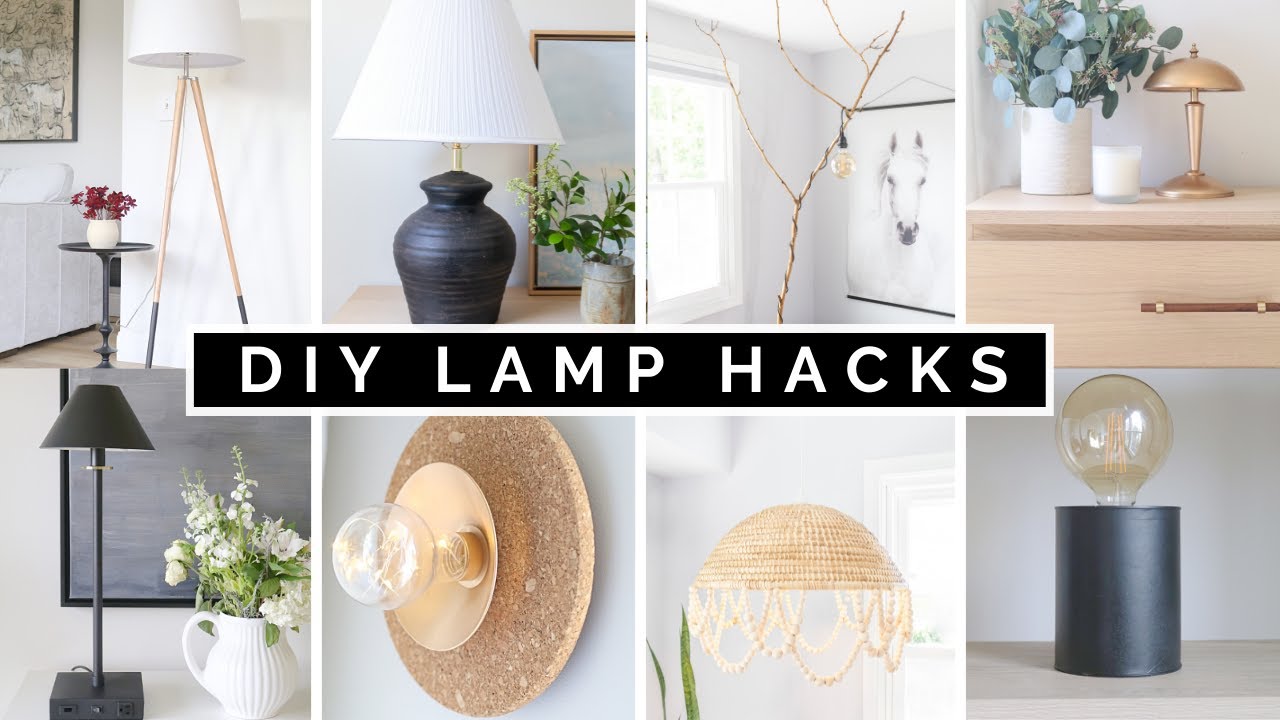The image appears to be an article from a magazine or an online platform showcasing DIY lamp hacks. Central to the design are the words "DIY Lamp Packs" in bold white letters set against a black background, flanked by a white border. The layout features eight distinct images of lamps arranged in two rows of four. Each image highlights a unique lamp style, offering inspiration for budget-friendly, creative lighting solutions. In the top left, there is a tall reading lamp in a room with white walls, accompanied by a flower on a stand. Next, a ginger jar lamp with a gray base and white shade. Adjacent is a lamp creatively draped over a tree branch in a living room. Completing the top row is a small gold desk lamp beside a plant-filled base. The bottom row starts with a simple light bulb in a black fixture, followed by a lamp with a woven rattan shade, a bare bulb attached to a cork background with a brass reflector, and a sleek black lamp with a unique round bulb. This collection of inventive lamp designs is presented in an elegant, accessible manner, appealing to those interested in DIY home decor projects.